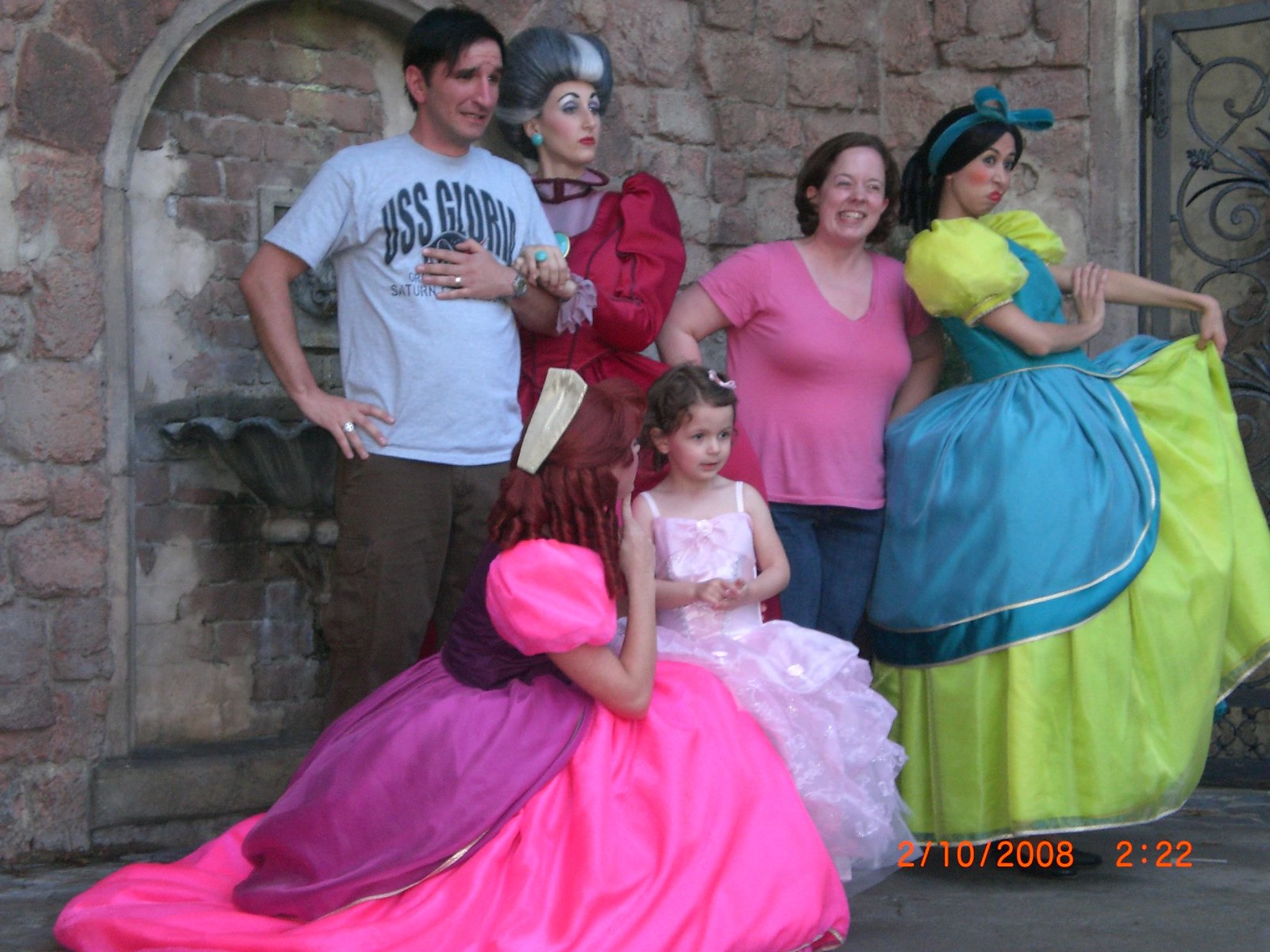In this charming photograph taken at what appears to be Disneyland or Disney World, a family of three—a mother, father, and their little girl—are posing in front of a stone wall adorned with a water fountain. The backdrop features the gray and pinkish hues of a Disney-themed castle wall. The mother, dressed in a pink t-shirt and blue jeans, and the father, sporting a white USS Glory t-shirt, stand on either side of the scene. The father, on the left, is making a distressed face as the evil stepmother from Cinderella, dressed in a striking red gown, holds his arm. To his right stands the mother, next to an evil stepsister in a yellow and teal dress with a teal bow, who playfully puckers her lips. The other evil stepsister, with red hair and a pink and maroon dress, crouches beside the daughter. The little girl is delightfully dressed in a light pink princess gown, reminiscent of Cinderella. The delightful chaos unfolds under a time stamp in orange, marking the moment as 2-10-2008 at 2:22 PM.